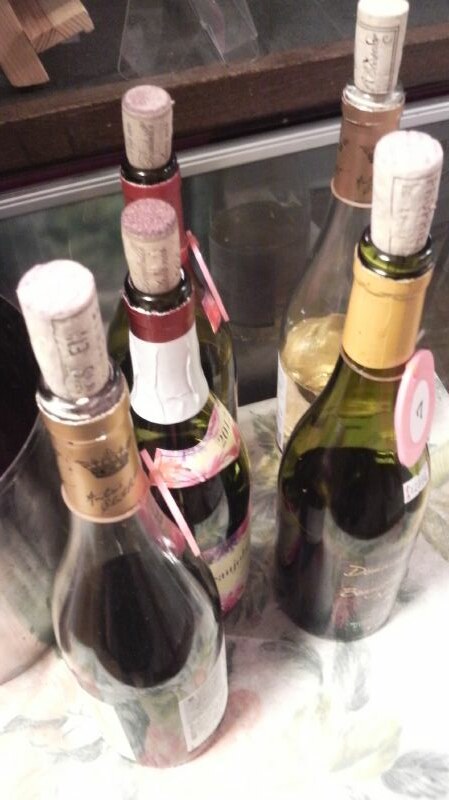This detailed photograph, taken from a slight upward angle, captures the scene of a white and grey (potentially marble) countertop. Prominently displayed are five open bottles of wine, each with a cork protruding from its top. These bottles vary in glass color—two green, two clear, and one indeterminate—and contain different varieties of wine: a mix of reds, whites, and possibly a Zinfandel, each with distinct red, gold, and white labels. All of the bottles are partially filled and arranged in a line with three centrally placed and two flanking the sides. To the left of the image, resting on the counter, there is a glimpse of a stainless steel pot, reminiscent of a spaghetti cooking pot. There is also a silver-metal bowl visible, partially within a glass container. In the background, there appears to be a wooden container adding a subtle rustic element to the overall modern setting of the image.